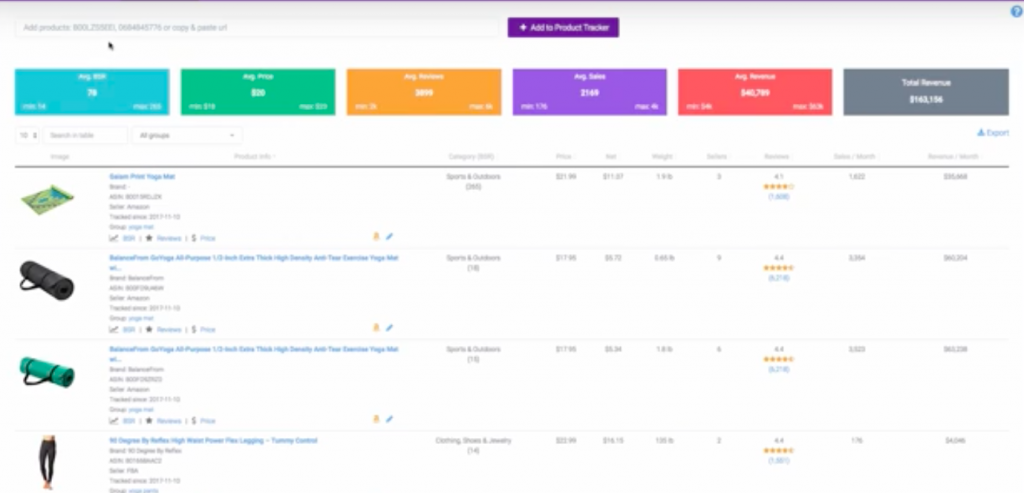This image depicts a cluttered web page featuring mostly illegible text. Prominently, a gray navigation bar spans the top, adorned with a thin, purple line above it. Within this gray bar, a search field is positioned on the left. Centrally located on the bar is a purple rectangle containing a drop-down menu.

Beneath the navigation bar, there are six rectangular buttons, each highlighted by distinct colors; from left to right, they are blue, green, orange, purple, red, and gray, with unreadable text within.

Following these buttons, the content is organized into sections with small, unclear headings and drop-down menus. The main section showcases several products. Each product listing includes an image on the left and a block of descriptive text, presumably detailing the product's features, pricing, and availability, on the right though this text is not legible.

The first product features a light and dark green yoga mat, laid out flat. Adjacent to it, the top line of text appears in blue, with black text beneath.

The second item is a black, rolled-up yoga mat equipped with a handle, flanked by blue text above and gray text below.

Next is a green, rolled-up yoga mat with a black handle, similarly accompanied by textual descriptions.

The last item displayed is a pair of black yoga pants, modeled from the waist down. This image also includes adjacent text detailing the product.